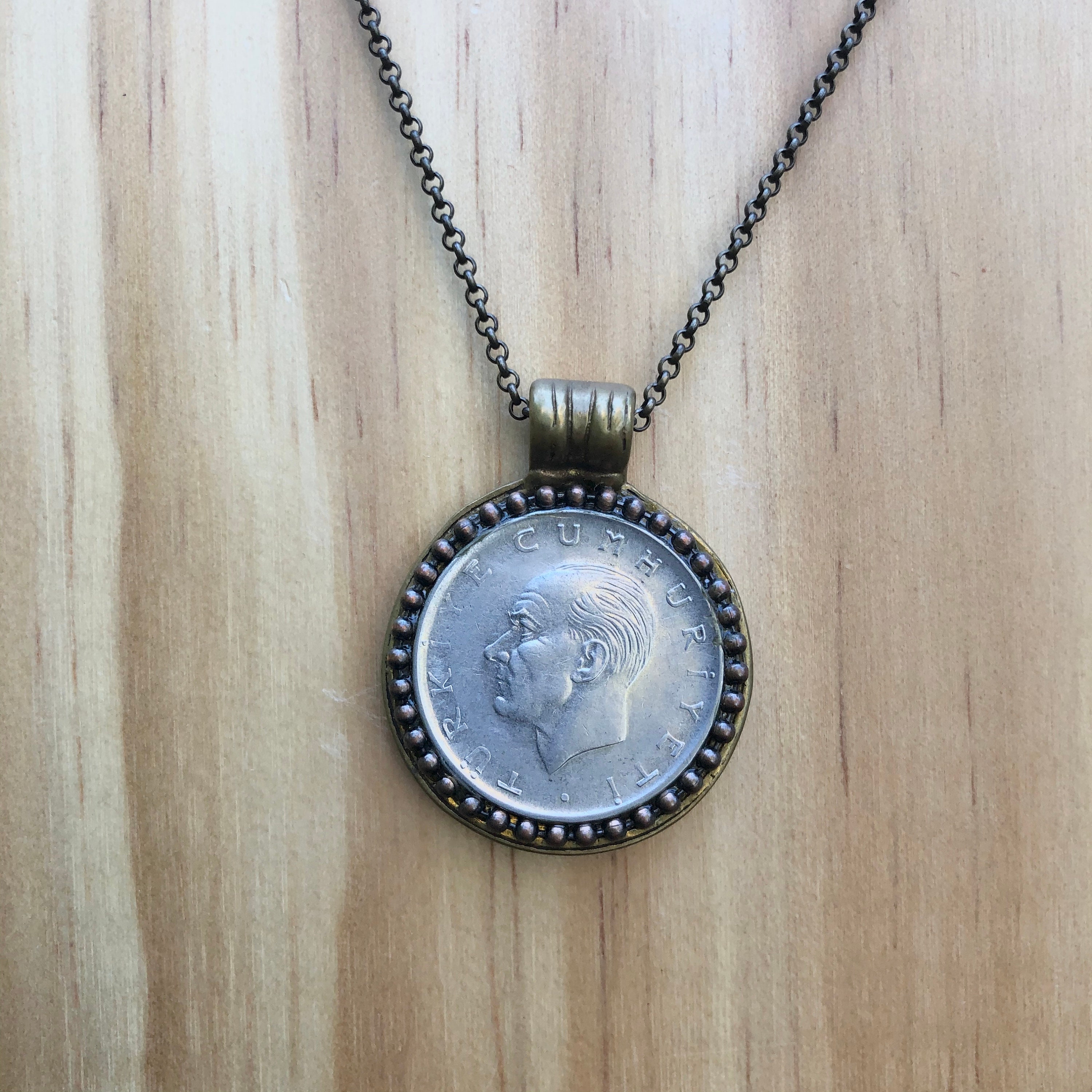This photograph showcases a distinctive pendant necklace, prominently displayed against a light tan wooden background. The pendant hangs from a dark beaded chain that extends from the top of the image to the center. The chain threads through a large, hollowed-out oval piece that appears to be silver. The pendant itself is round, framed by evenly spaced small copper or bronze beads along its perimeter. At the top of the pendant, a goldish-bronze clasp attaches it to the chain. Engraved within the circular pendant is the profile of a balding man with short hair, accentuated by raised details. Surrounding the man's profile is text in an unfamiliar language, reading "Cumhurt Yeti Turk," suggesting it might be a Turkish coin or medal.